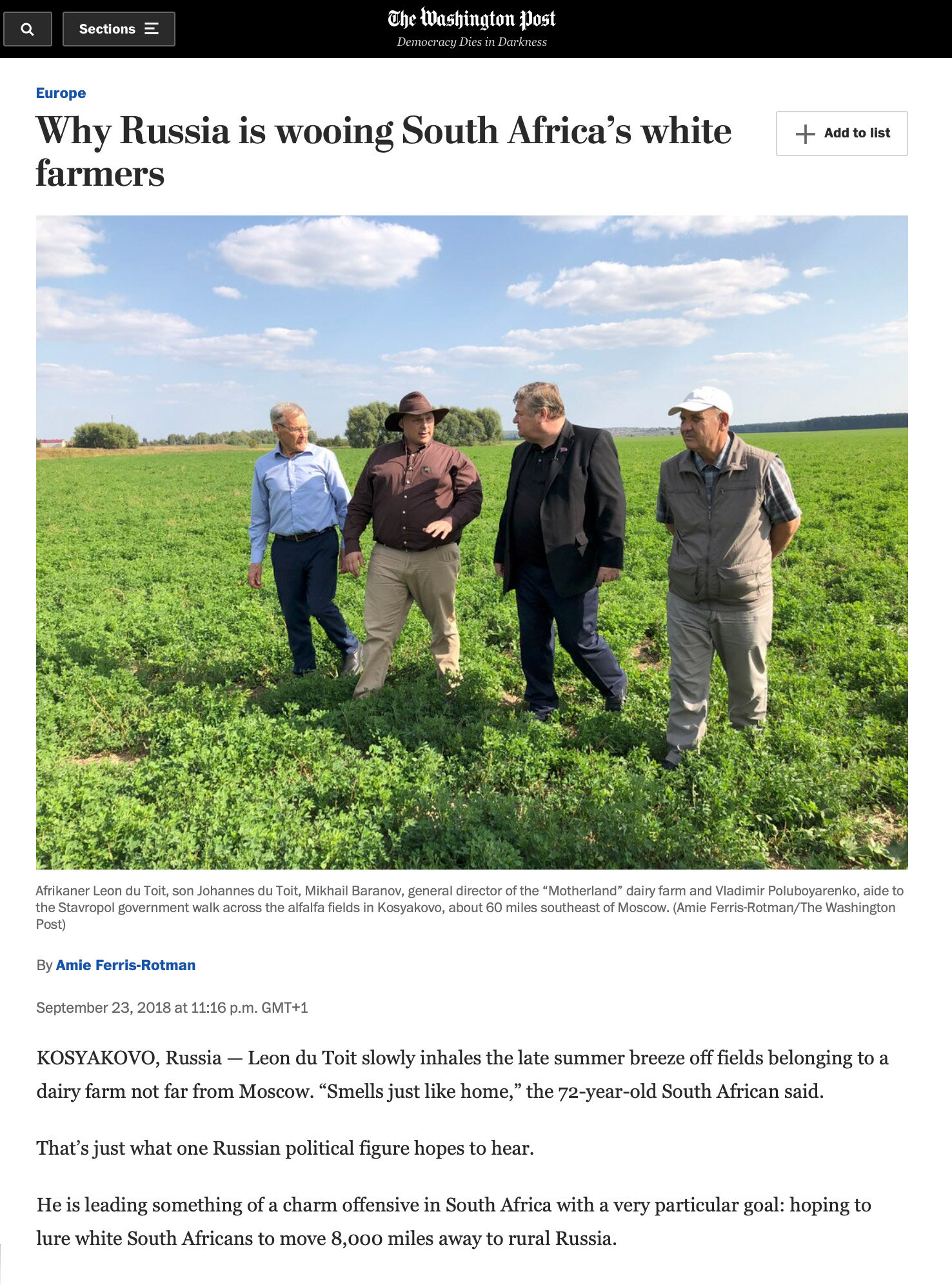This image features a detailed article header from "The Washington Post." The top part is a black border extending across the image. On the left-hand side, there's a black rectangle with two outlined white icons: the first icon depicts a white magnifying glass, and next to it, there is a white rectangle with three lines labeled "Sections." In the center of this border, "The Washington Post" is written in white, accompanied by the slogan "Democracy Dies in Darkness." The background is white, with a blue heading on the left that reads "Europe." Below the heading, in black text, is the article title: "Why Russia is attracting South Africa's white farmers."

Beneath the text is an image showcasing a landscape with a brilliant blue sky dotted with white clouds, vibrant green grass, and four individuals identified as white, standing on farmland. There is lush greenery stretching towards the horizon. 

A detailed caption under the image reads: "Akhenaten Leon Dutoy, son of Joannes Dutoy; Mikhail Baranov, general director of Motherhood Dairy Farm; and Vladimir Poluboy Garnano, aide to the Stavropol government, walk across the alfalfa fields in Kostkovo, about 50 miles southeast of Moscow."

The author's name, "Amie Ferris-Rotman," is printed in blue beneath the image, followed by the date and time of publication in black: "September 23, 2018 at 11:16 p.m. GMT+1."